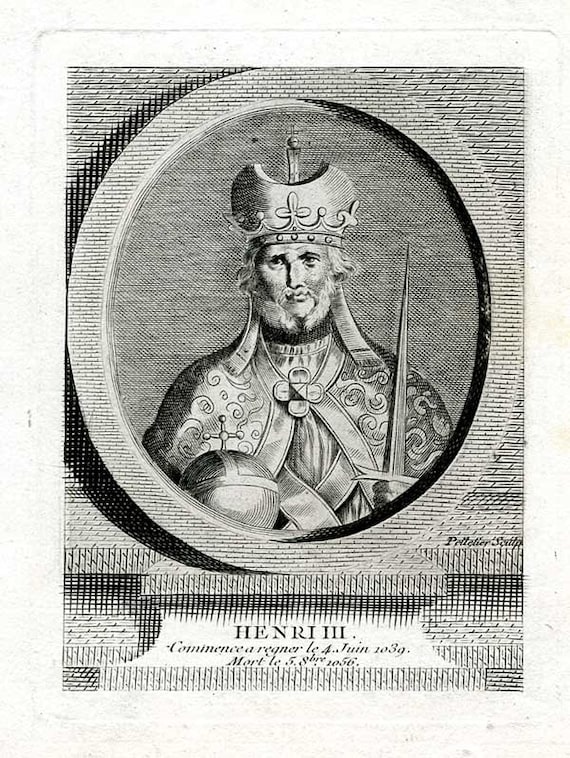This is a black and white illustration of King Henry III. He is depicted from the chest up, wearing an ornate crown with a crescent moon-shaped hooded crest on top, and a small pillar with a ball and cross. His regal attire includes elaborate robes fastened with a large clover-shaped seal. In his left hand, he holds a short, pointy sword, and in his right, he holds another object that appears to be a scepter or helmet. Henry III, who has a full white beard and looks somber, is framed within an oval border that resembles tiny bricks. Below the portrait, the text reads "Henry III" in bold, followed by a script that likely signifies significant dates: "commence, arraignar, le 4 juin 1039; mort, le 5 avril 1056." This detailed depiction bears resemblance to a grave marker or a historical commemoration underlining his reign and death.